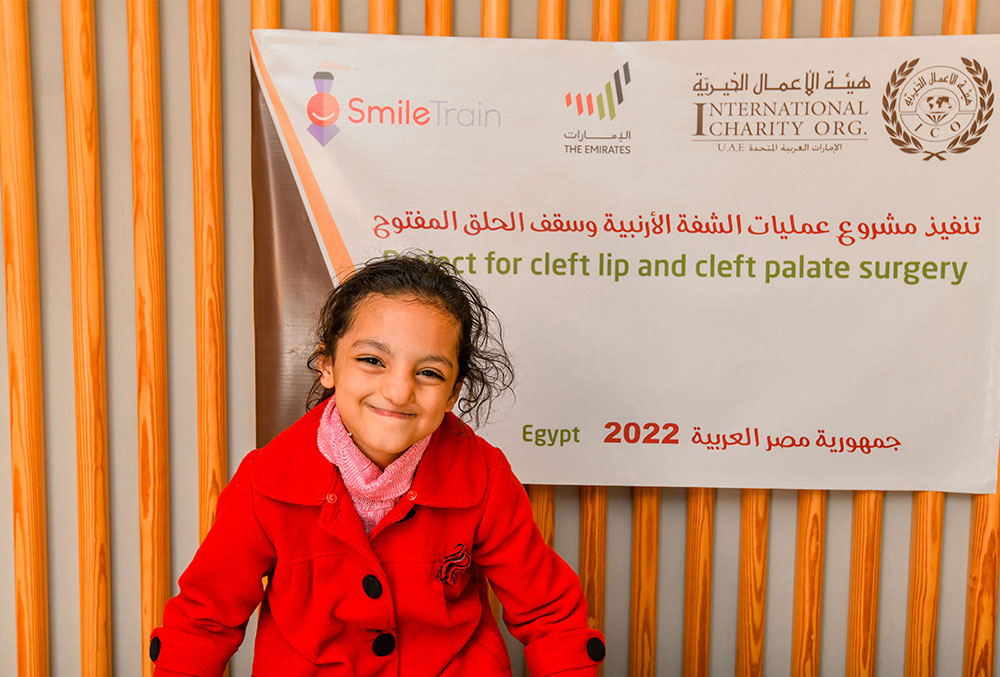The photograph features a young girl with light brown skin, smiling with her mouth closed, her head tilted slightly to the right. She has somewhat messy black hair and is wearing a warm red coat with large black buttons, paired with a pink scarf underneath. Positioned slightly to the left of center in the image, she is visible from the torso up. Behind her, there is a grayish-blue wall adorned with several orangey-brown wooden poles stretching horizontally, creating a textured background. Just above her left shoulder and extending to the right side of the photograph, a sign is prominently displayed. The sign, on a piece of paper, includes the following text: “Smile Train,” featuring a logo with a smile and a triangle resembling a train. Below this, it reads, “International Charity Org,” and further details indicate, “Perfect for Cleft Lip and Cleft Palate Surgery, Egypt 2022.” The girl’s joyful expression and attire suggest she may be a beneficiary of the mentioned surgery program.